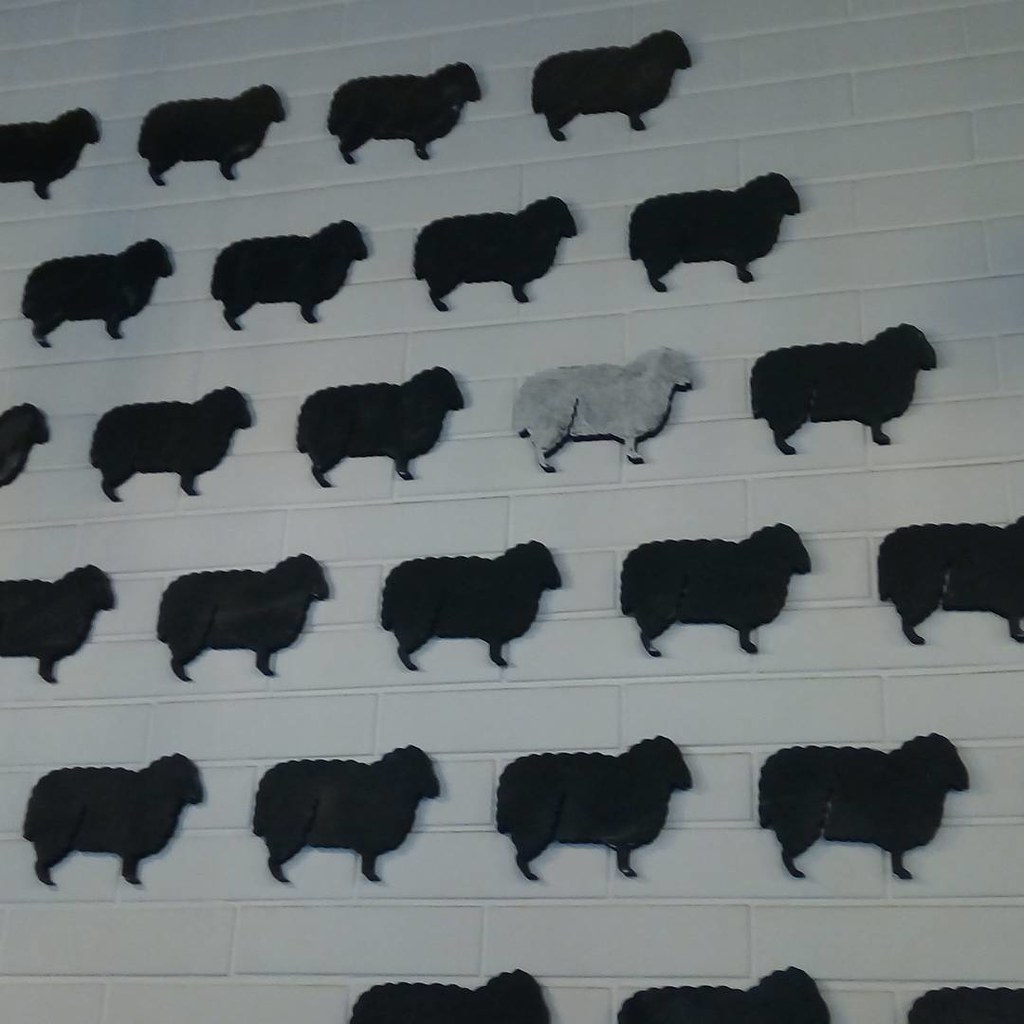This is a vertical rectangular photograph depicting a white brick wall adorned with small, decorative sheep cutouts. Despite the monochromatic black-and-white presentation, the details of the image are clear. There are six staggered horizontal rows of 25 sheep arranged in an offset pattern, all facing the right side of the photograph. Most sheep are black, but there is one distinctive white sheep situated in the third row, second from the right. The first row comprises four black sheep, with the first one partially cut off by the left edge. The second row also features four black sheep. In the third row, a partially cut-off black sheep is followed by a grayish-white sheep and another black sheep. The fourth row has five sheep, with the first and last cut off by the image edges. Four black sheep make up the fifth row. The final row displays three sheep, but only their tops are visible as they are cut off by the bottom edge. The staggered arrangement, the white brick's texture, and the perspective, which causes the top rows to tilt slightly upward, contribute to the simple yet detailed composition of the image.